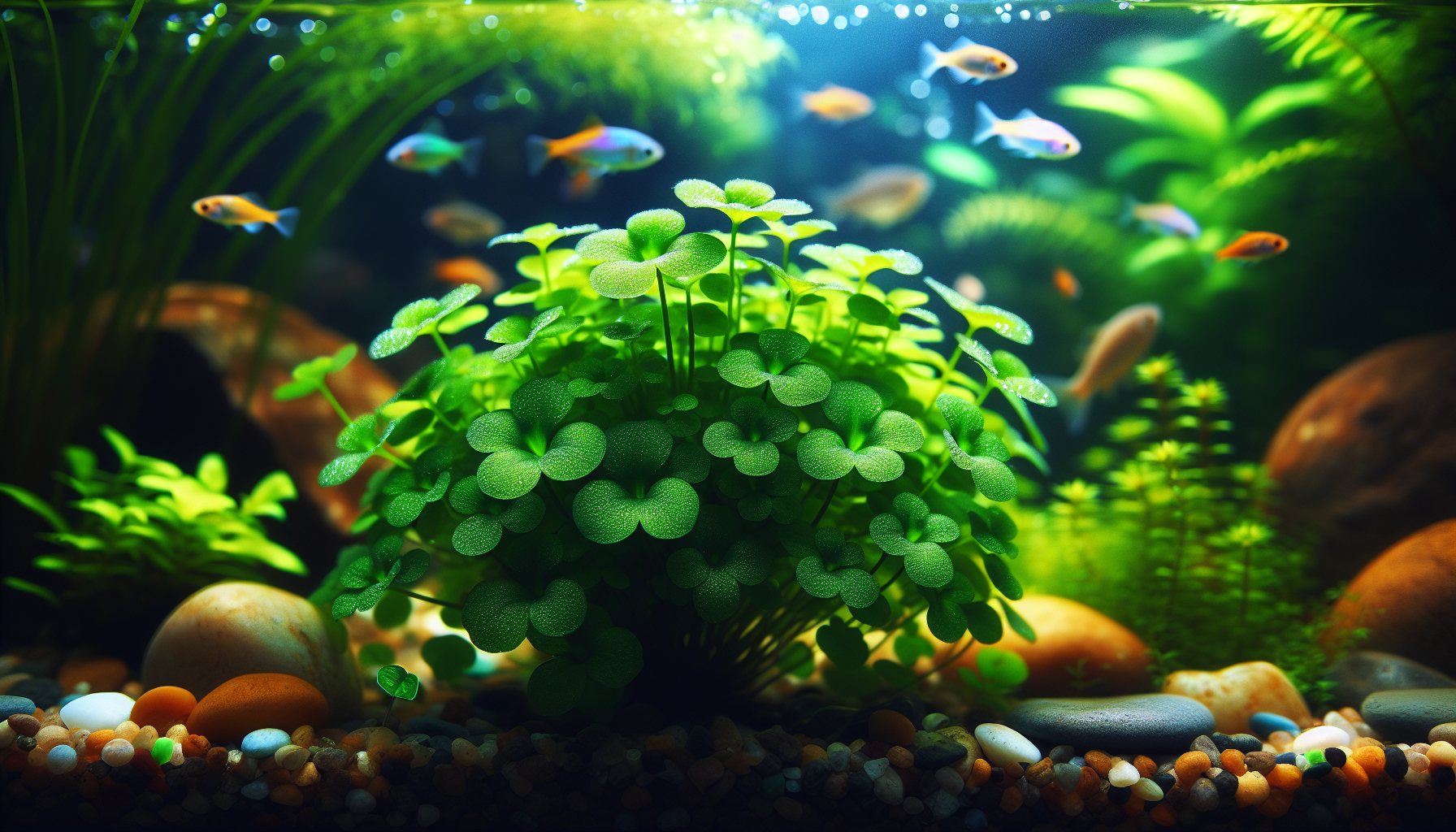This high-definition image captures the interior of a vibrant fish tank. The tank's floor is adorned with a diverse array of pebbles in greens, blues, browns, oranges, and whites, with sizes ranging from small to very large. Front and center, a distinctive green plant resembling clover takes prominence, flanked by taller, slankier green plants on the left and a fern-like plant in the background to the right. Scattered throughout the tank, a variety of small, colorful fish swim about; their bodies showcasing vibrant hues of orange, gray, purple, green, and pink. Some of these fish are clearly visible and sharply defined, while others appear more blurred in the background, adding to the depth of the underwater scene. Bubbles rise gently to the top, emphasizing the lively, aquatic environment.